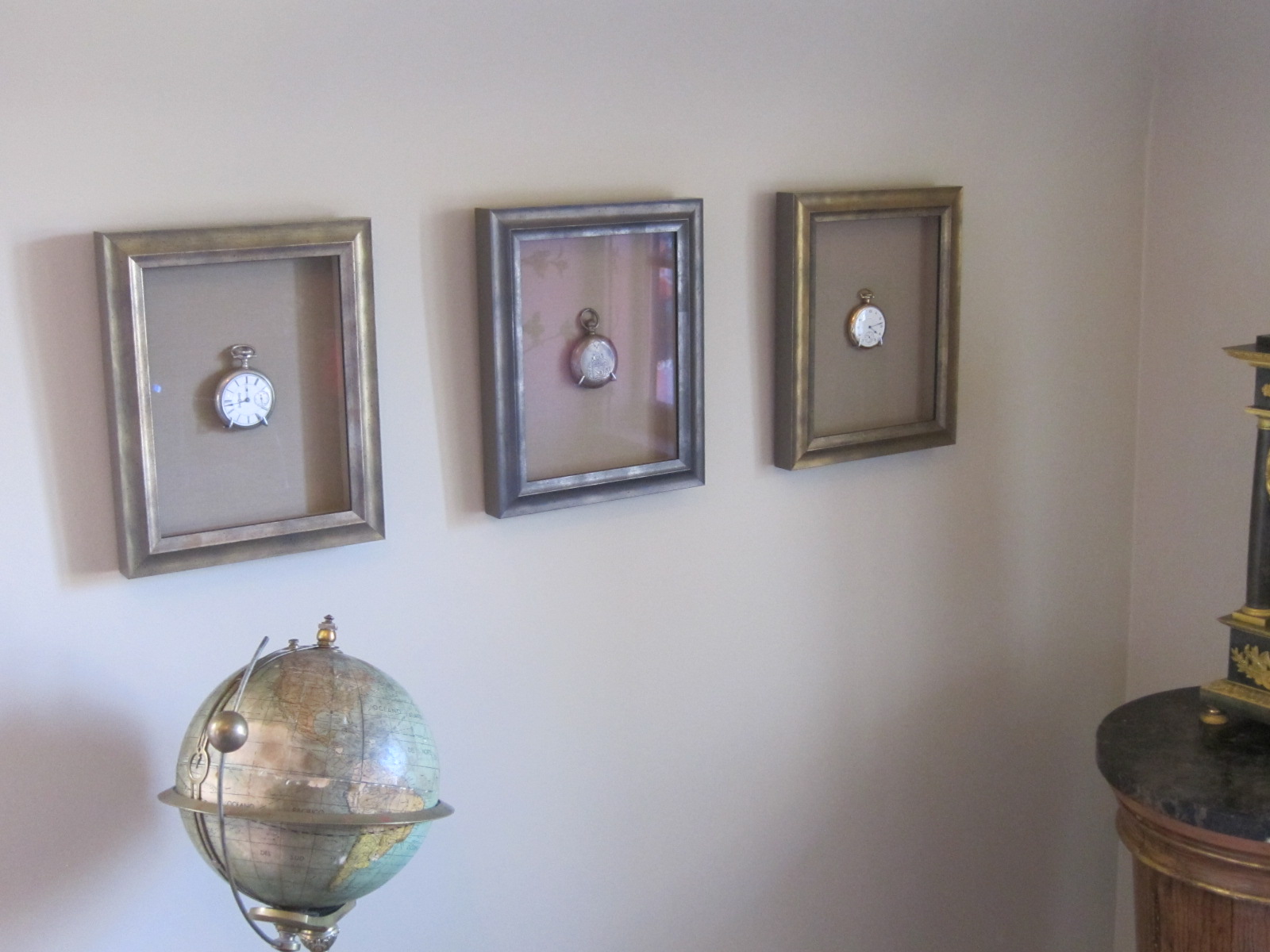This image depicts a section of a white, smooth wall adorned with three horizontally aligned picture frames. Each frame contains a vintage pocket watch, emphasizing the wall's antique aesthetic. The first frame on the left is silver, housing a pocket watch with a white face and black numbers. The middle frame is a dark gunmetal silver, showcasing another classic pocket watch. The frame on the right is golden, encasing a pocket watch with a white face and black ticks. In front of these frames, an old-style globe with predominantly greenish hues sits on a stand, adding to the nostalgic ambiance. On the bottom right of the image, part of a small table with a black marble-like surface is visible, topped by what appears to be a miniature clock tower with gold legs.